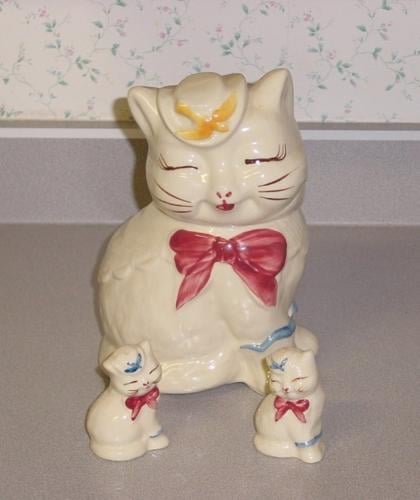The image showcases a trio of porcelain cat figurines displayed on a grey table, possibly a kitchen counter. The set includes one large mother cat and two smaller kitten cats. All three figurines are cream-colored with painted details. The mother cat features a closed-eye expression, a red bow tie, and a pink hat adorned with a yellow bird on top. The two kittens, both wearing blue ties, have similar closed-eye expressions and red bows. The backdrop is a white wall decorated with a floral pattern in green and yellow tones. The overall setup suggests a decorative ensemble that could be part of a collection.